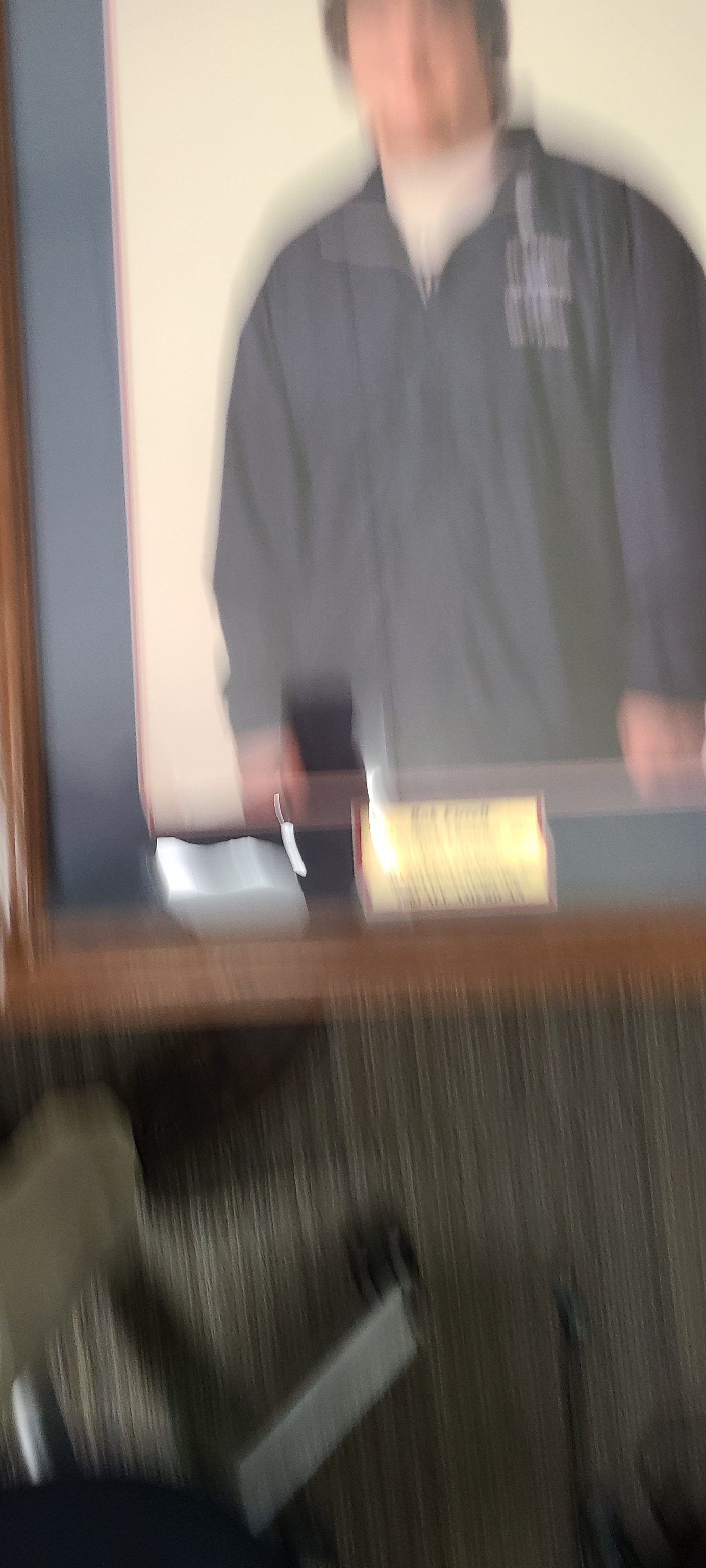This image features a blurred scene dominated by a central horizontal wooden picture frame. The frame appears to hold a portrait of a man. The man in the photograph has brunette hair and is wearing a blue vinyl pullover over a white turtleneck. The left lapel of his pullover has some writing on it, though the text is not legible due to the blur. Below the frame, there are several vertical lines stretching across the width of the image, resembling the strands of a wig, though it is not actually a wig.